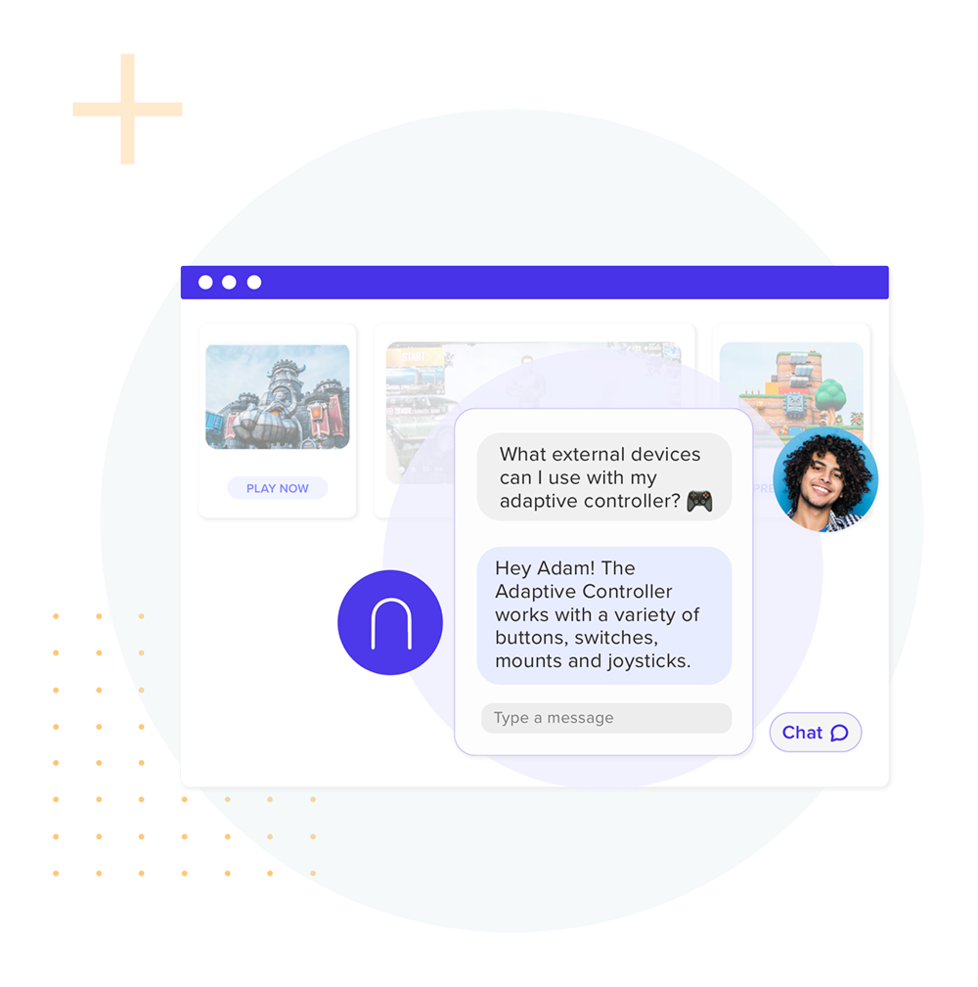This image appears to be a screenshot from a computer interface. The background is predominantly white with a subtle, light gray circle in the center. In the upper left corner, there is a noticeable yellow plus sign. Toward the bottom right corner lies a grid of dots, arranged in an 8x8 square configuration.

Central to the image is a pop-up screen. The pop-up is framed by a blue border along the top edge, featuring three white circles clustered in the left corner. Within the left section of the pop-up, there is a smaller rectangle depicting an outdoor scene with some buildings, accompanied by a "Play Now" button.

Dominating the center of the screen is another pop-up that displays a text conversation, suggesting it may be a chat function. The chat text reads: "What external devices can I use with my adaptive controller?" followed by a controller emoji. Below, a response is visible: "Hey, Adam, the adaptive controller works with a variety of buttons, switches, mounts, and joysticks."